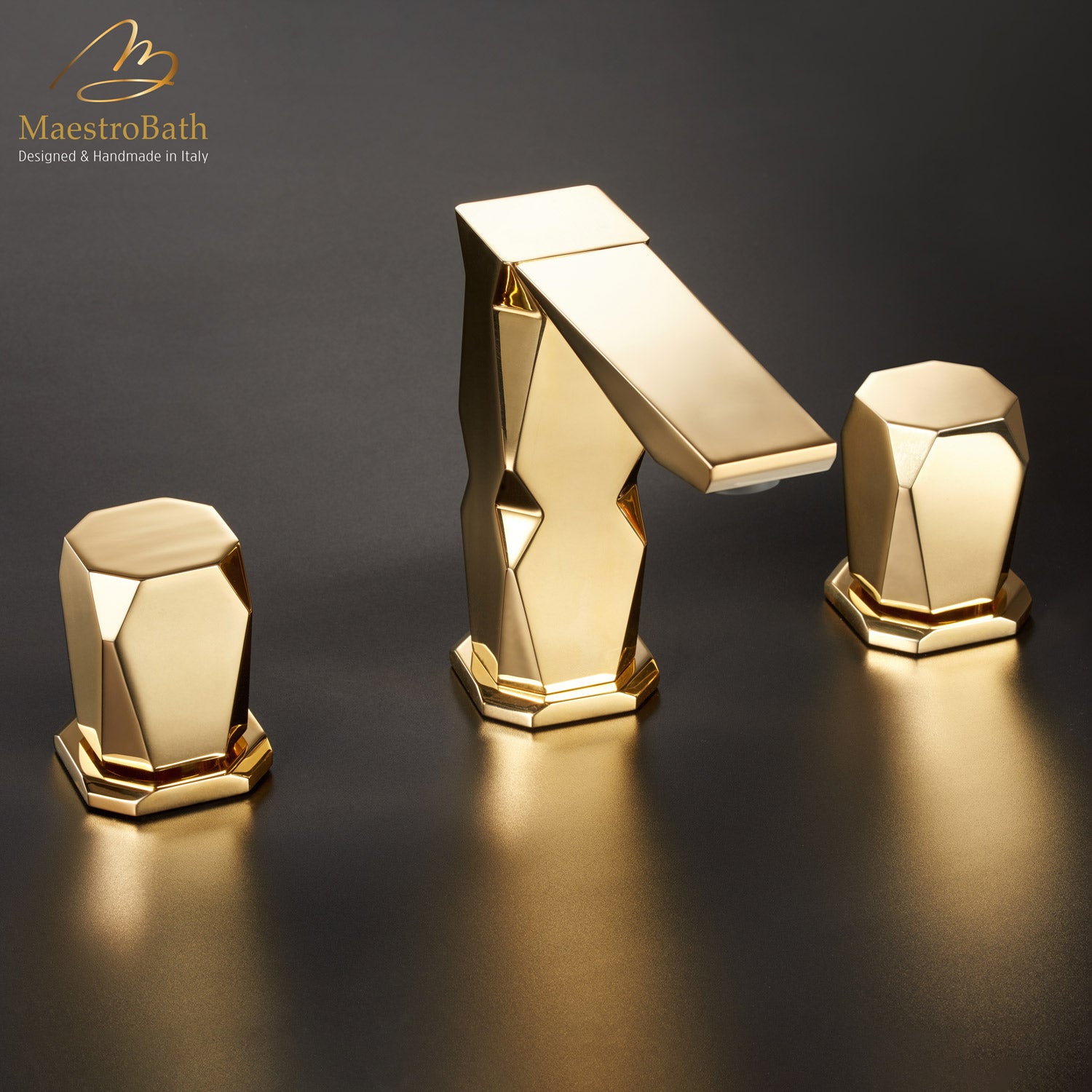This advertisement features a luxurious, high-end modern faucet set against a sophisticated dark gray background with subtle dark spots. The center of the image is dominated by the main spout, crafted in an exquisite gold hue. The spout is designed with a unique, organic crystal-like form, featuring various polygonal faces that create an intricate, multifaceted appearance. The water outlet is a sleek, flat, and thin rectangular shape, enhancing the modern aesthetic.

Flanking the spout are two separate knobs for controlling the water flow. These knobs share the same crystalline design as the spout, composed of intersecting geometric shapes that contribute to a cohesive and elegant look. Each knob sits on a refined gold, copper, and bronze base, and their reflections can be seen on the dark gray surface below, adding a touch of visual depth and sophistication.

In the top left corner, a golden cursive "M" is prominently displayed, symbolizing the brand's identity. Below it, in gold lettering, is the brand name "Maestro Bath," and beneath that, in smaller white text, are the words "Design and Handmade in Italy," emphasizing the craftsmanship and bespoke nature of the product.